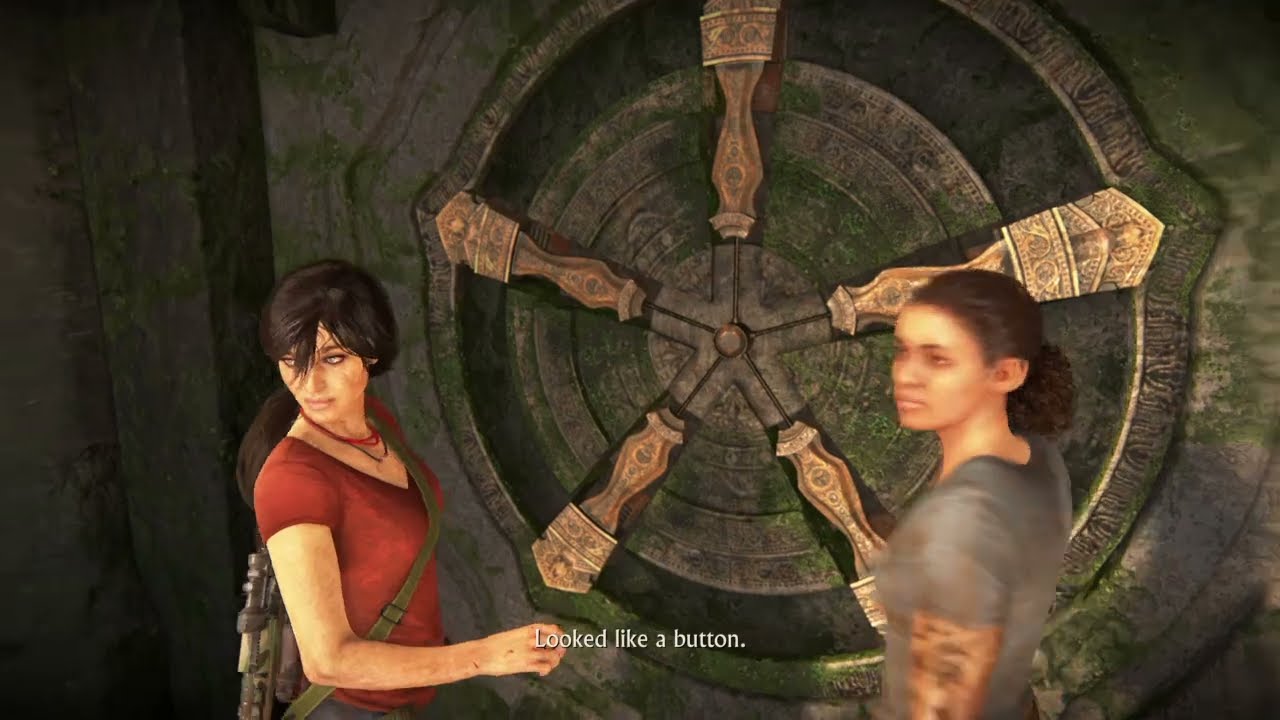This image appears to be a screenshot from a video game reminiscent of titles like "Uncharted" or "Tomb Raider," featuring a detailed scene with two female characters in a 3D-rendered environment that suggests a graphical style common between 2017 to 2020. On the left, a woman with long brown hair tied in a ponytail, tan skin, and a red short-sleeved shirt is seen. She has a green strap over her shoulder, holding a large silver gun, and is also wearing some necklaces. The woman on the right seems to be a Black woman with curly brown hair tied back into a bun. She has tattoos on her arm, is wearing a gray short-sleeved shirt, and has her gaze directed to the left. Both women stand in front of an elaborate stone wall covered in green moss. At the center of this wall is a large, circular mechanism that resembles a complex vault or puzzle. The circular piece features a central point with radiating lines forming a star-like pattern and includes tan-colored pillars that suggest they may slide up or down. The bottom of the image displays text reading "look like a button." This scene likely depicts a moment where the characters are trying to solve a puzzle to gain entry through the vault-like door.